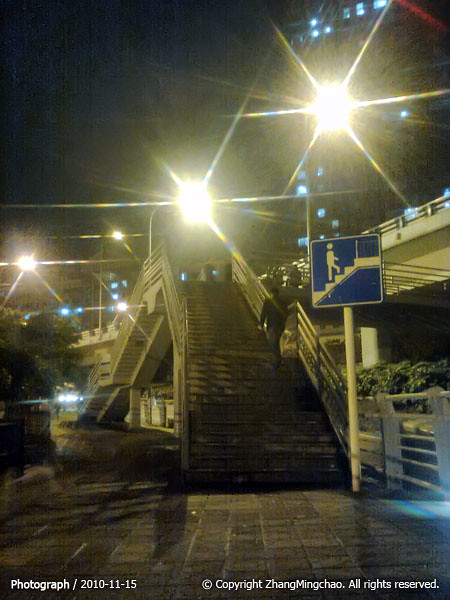This nighttime image captures an outdoor staircase beside an overpass or bridge, illuminated by bright spotlights lining the structure above. In the center of the photo stands a multi-flight staircase extending upwards, bordered by a white fence along the sidewalk flanked by trees and bushes. A blue sign on a white pole near the base of the staircase features an icon of a person climbing stairs. A man can be seen ascending the steps, which lead from a dark, dirty-brick ground. The backdrop includes a tall, light-emitting skyscraper, though details are obscured by glare. Text in the lower left corner of the image reads, "Photograph, 2010, 11, 15. Copyright, Zhang Mingchao."